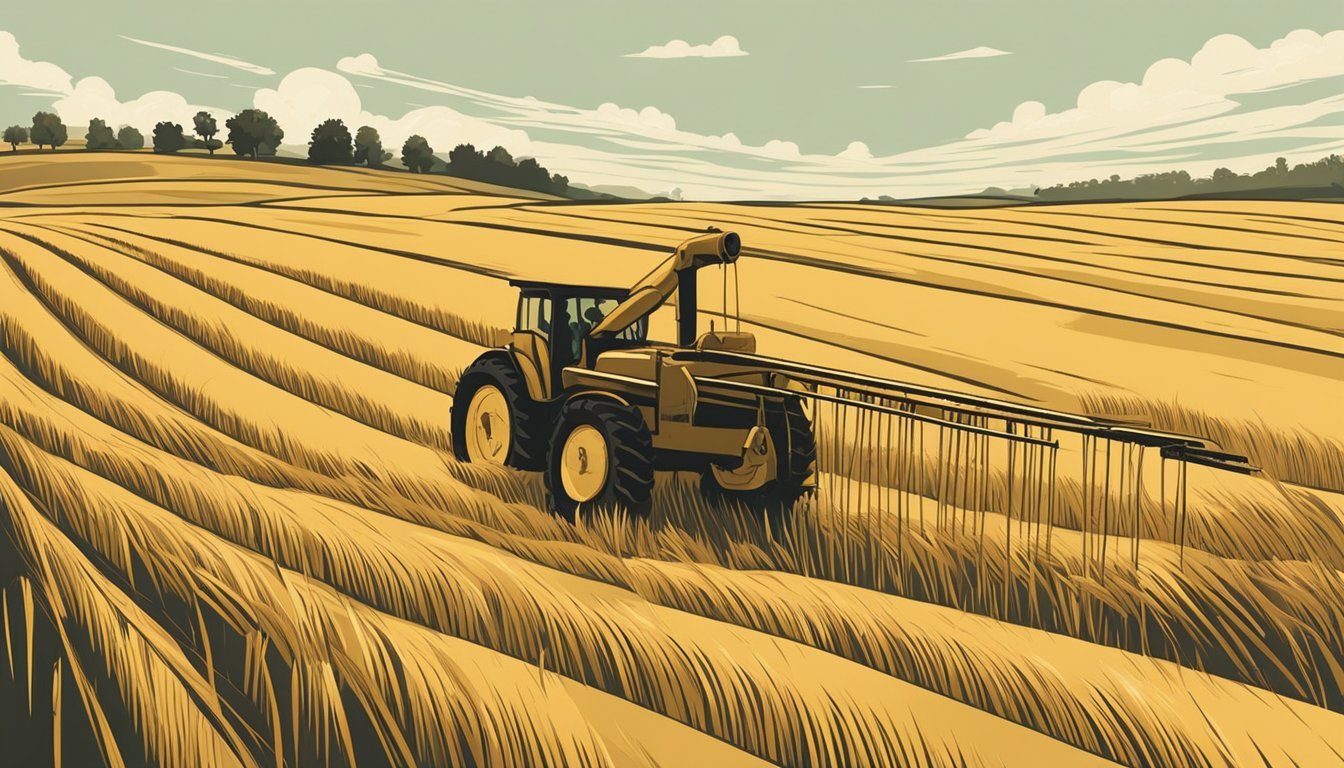The illustration is a highly stylized drawing, potentially an oil painting, depicting a vast farmland scene. The yellowish-beige crop, likely wheat or hay, is meticulously organized in rows across gently rolling hills. Dominating the foreground is a large, light yellow tractor with four massive black tires and a covered cab. Attached to the front of the tractor is a long implement, possibly a combine or harvester, with what appears to be hay or grain hanging from its bottom, indicating an active harvesting process. The background features an olive sky with wavy, swirling clouds and a line of green trees, suggesting a natural and serene landscape. The overall color palette primarily consists of sepia tones, contributing to the vintage, artistic feel of the image.